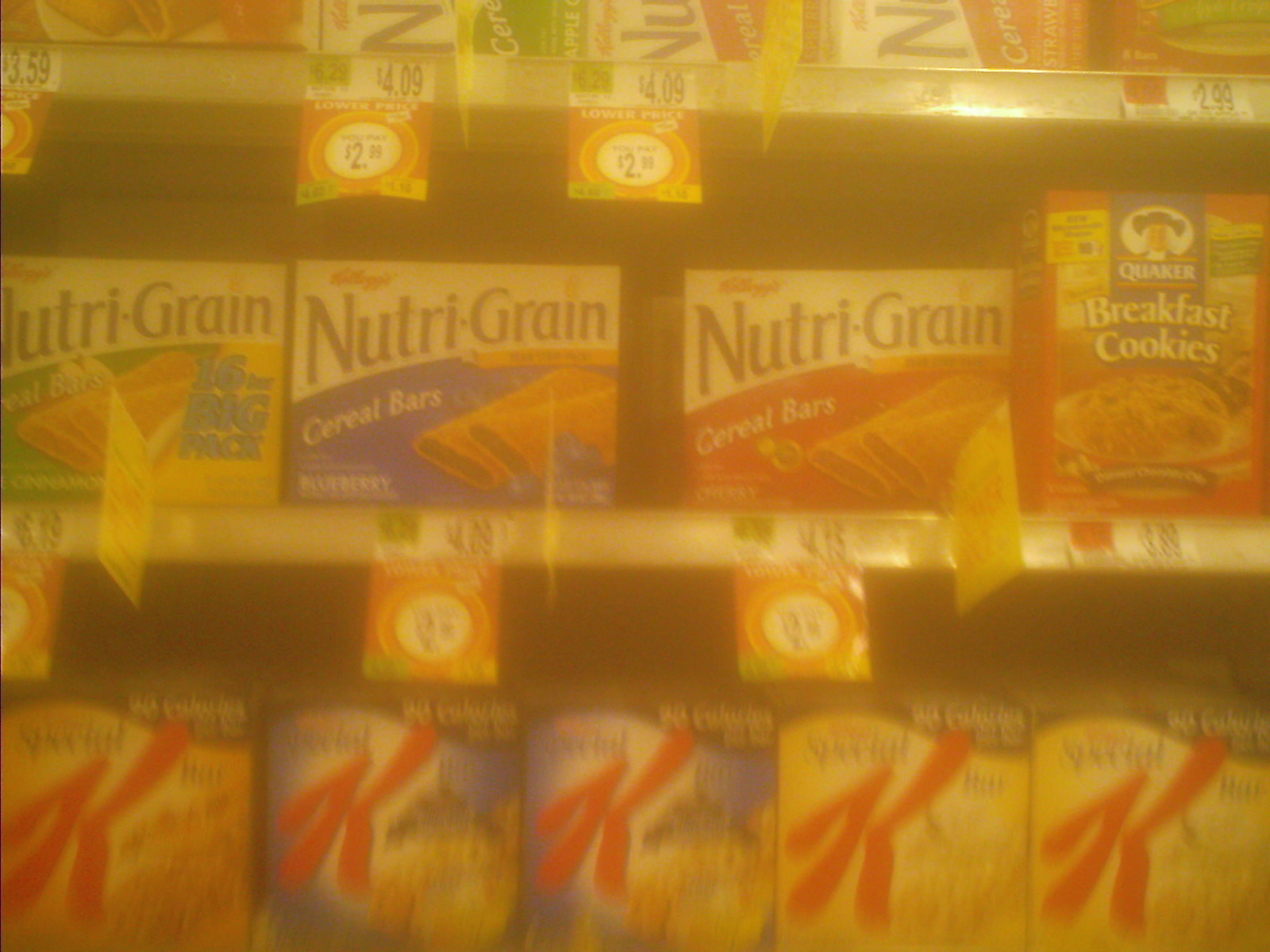The photograph captures the vibrant interior of a grocery store, specifically focusing on the breakfast aisle. The shelves are stocked with a variety of breakfast products, highlighting an array of Nutri-Grain bars and cereals. Prominently displayed on the middle shelf are three boxes of Nutri-Grain cereal bars in green, purple, and red boxes, likely representing apple, blueberry, and strawberry flavors respectively. To the right, there is a box of Quaker breakfast cookies, which seems to depict a type of oatmeal in a bowl on its packaging.

Beneath these, a row of five boxes of Special K cereal is visible, each a different variety and color, including yellow and purple boxes. On the top shelf, more Nutri-Grain items can be seen, although they are partially obscured, revealing only "NU" on the packaging. The price tags show a range from $4.09 to $3.99 and $2.99. 

The photograph itself is slightly overexposed, casting an orange glow across the scene, and is notably blurry, detracting from the clarity of the details.